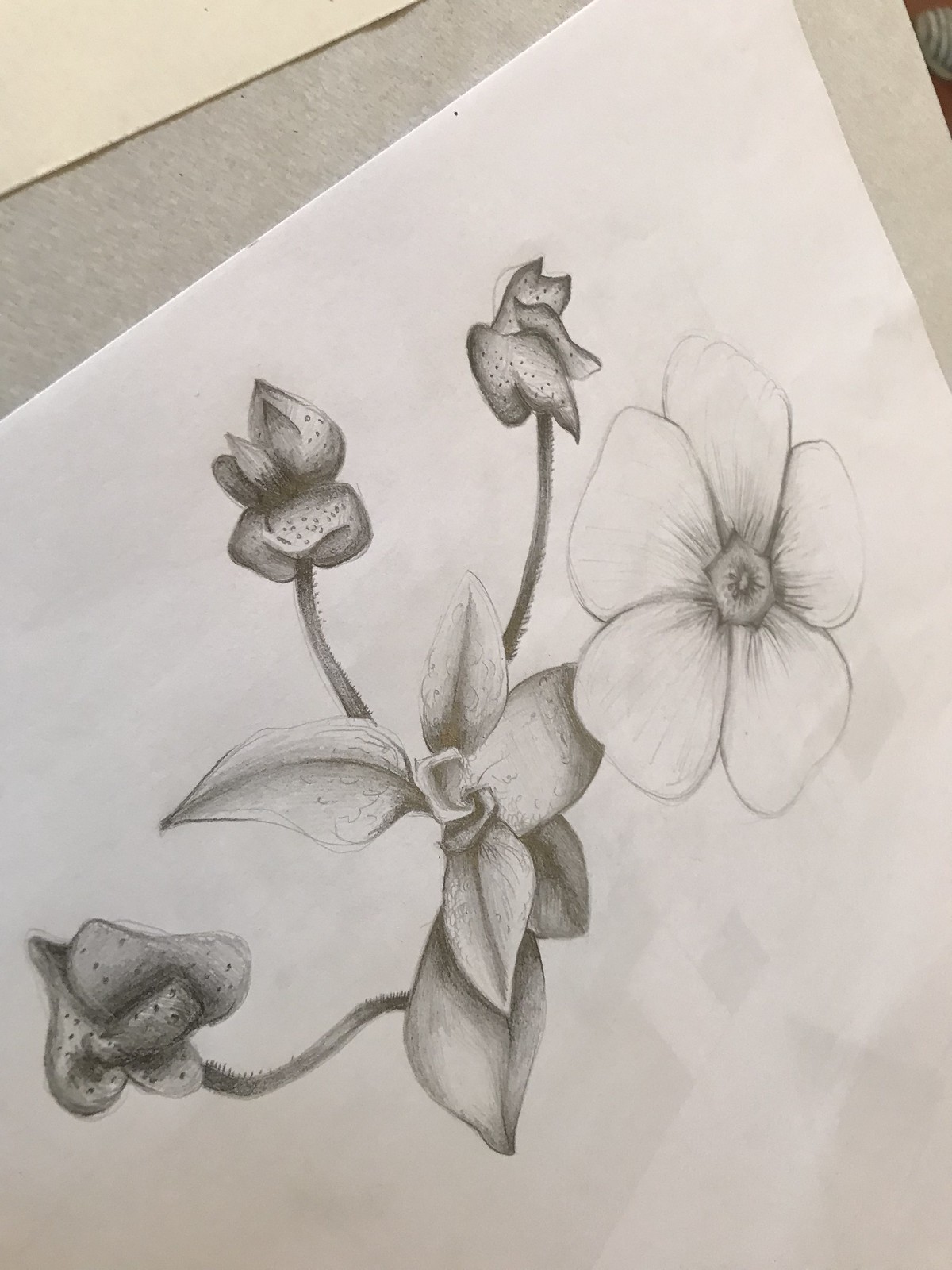The illustration depicts a white flower prominently positioned on the right side of the image, set against a diverse backdrop of various fabrics. The petals of the flower are detailed with intricate dark speckles, creating a stark contrast against their white base. The center of the flower is skillfully shaded, featuring subtle curves that add a sense of depth and realism. On the leftmost part of the flower, the shading includes small dots, further enhancing its textured appearance. The stems, slightly fuzzy with defined edges, extend gracefully from the base of the flower, leading into large, lush leaves that support the delicate bloom. The combination of the fabric background, the textured petals, and the detailed shading comes together to create a visually striking and rich illustration.